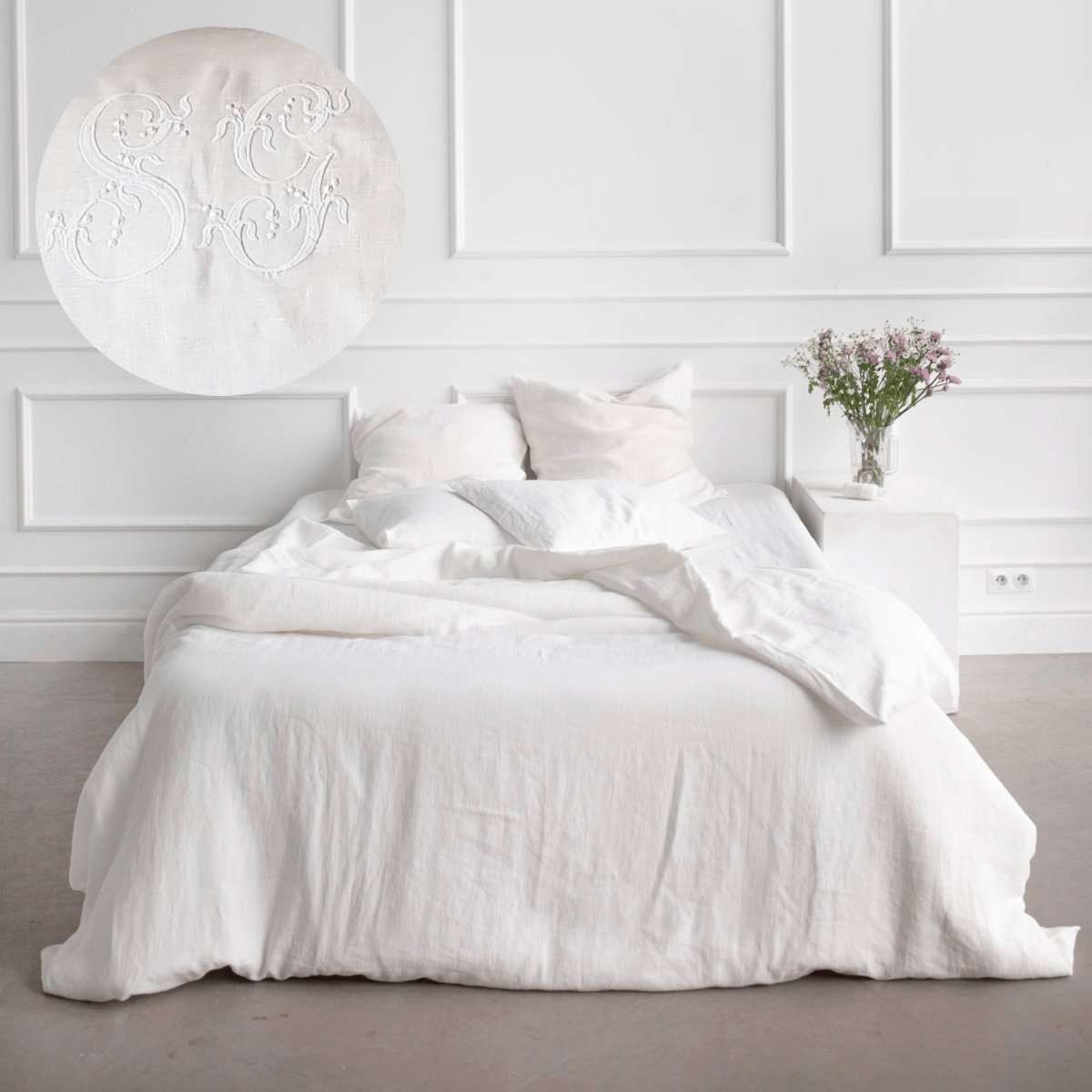This image captures a section of a predominantly white bedroom, potentially part of a furniture showcase. Dominating the scene is a centrally placed queen-size bed, dressed in white sheets, with two white pillows and an additional set of two white pillows laying on top. The bed linens are somewhat disheveled but not completely untidy. Adjacent to the bed, on the right, stands a simple, rectangular nightstand at the same height as the bed. This nightstand holds a vase containing flowers with green stems and pink and white blooms. The room's flooring appears to be a tan or light gray concrete tile. 

Behind the bed, the white wall features a design with raised square and rectangular panels, interrupted only by a wall outlet visible on the right side. In the upper left corner of the image, there is a circular, cloth-like object with the initials "SG" stitched in fancy lettering. No people or animals are present in the picture, highlighting a serene and immaculate bedroom setting with accents of green and pink from the flowers and a hint of tan or gray from the floor.